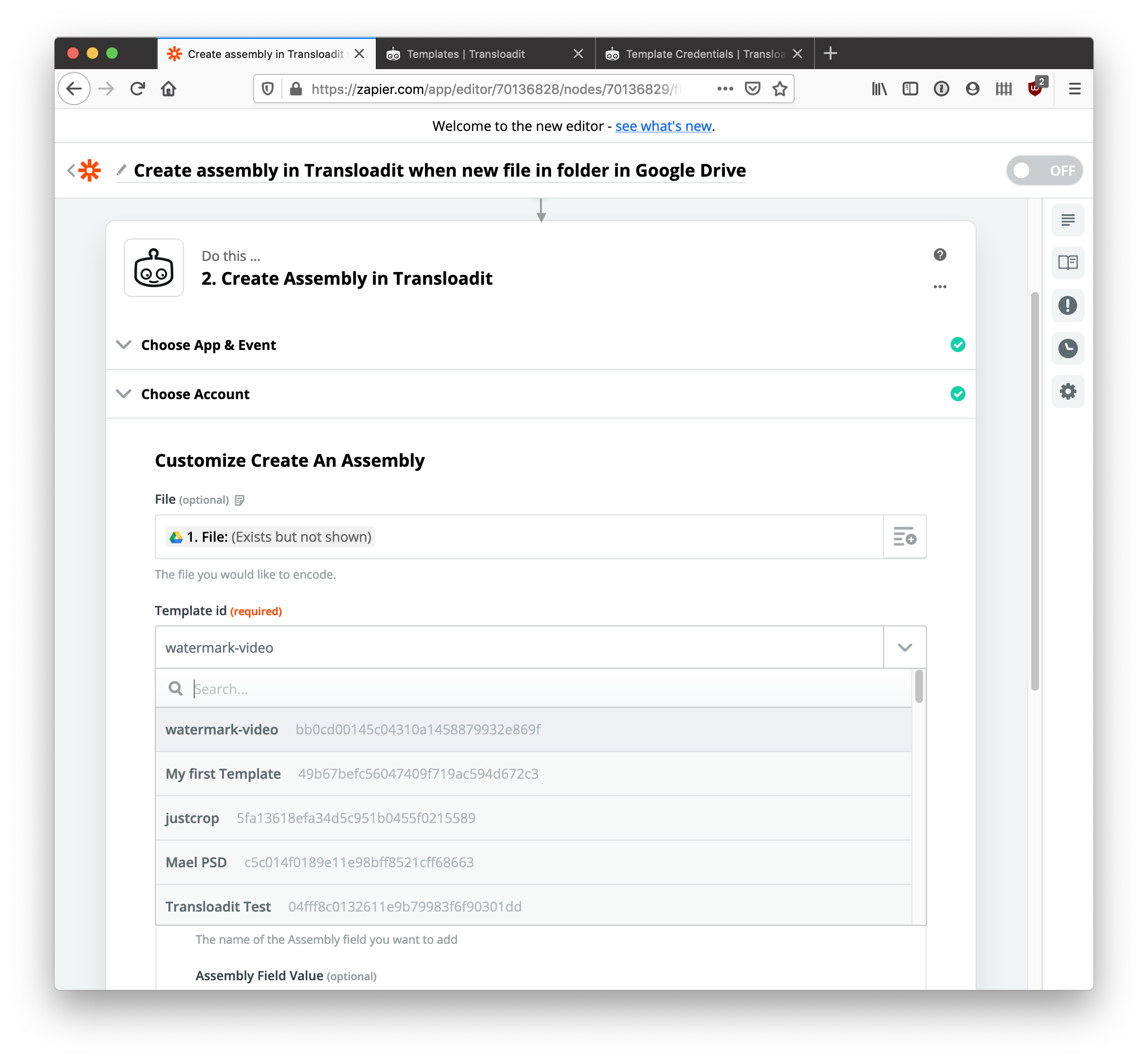This image captures a portion of a website displayed in portrait mode, specifically showcasing a form within the Zapier platform. In the upper left-hand corner, there are three dots—red, yellow, and green—set against a black background, typical of the standard Mac window control buttons. 

Adjacent to this is a highlighted white tab that reads "Create Assembly in Transload IT." Below it are two black tabs labeled "Templates, Transload IT" and "Template Credentials." 

The main form begins with a white background area that includes a search bar at the top, displaying the URL "zapier.com/app/editor." The next row underneath features a welcoming message, "Welcome to the New Editor," followed by an underlined light blue hyperlink stating, "See what's new."

Continuing down, there's a descriptive row that says, "Create assembly in Transload IT when new file in folder in Google Drive," accompanied by a toggle switch currently in the 'off' position.

The form is structured into multiple segments. Under "Do This," the first step is to "Create Assembly in Transload IT." The following row, "Choose App and Event," is marked with a green checkmark, indicating completion. The subsequent row, "Choose Account," also has a green checkmark. The next section, "Customize Create an Assembly File," starts with a prompt, "File Exists but Not Shown," requesting the user to specify the file they wish to encode. Additionally, a field marked with "Template ID" in red indicates it is required. 

Within this section are various options for template selection, such as "Watermark Video." There is a search bar below this for further specification, followed by five selectable template options listed as "My First Template," "Just Crop," "Just Crop," and "M-A-L-L," allowing the user to choose one of these.

Overall, the form is detailed and organized, guiding the user through the process of setting up an assembly operation in Transload IT via Zapier.